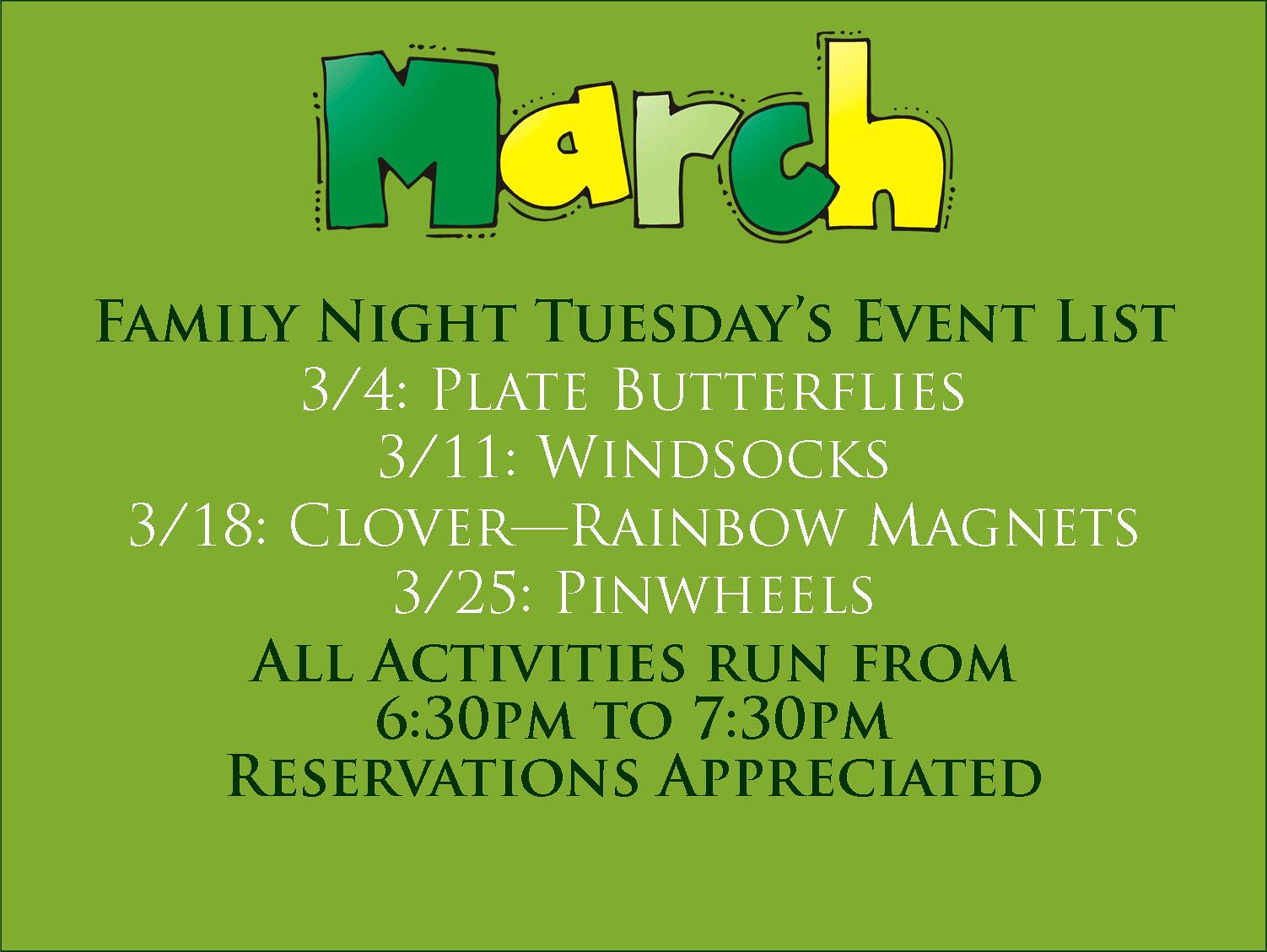The advertisement is a colorful and lively flyer promoting a series of Family Night events held on Tuesdays in March. The background is a vibrant green, and at the top center of the flyer, the word "MARCH" is depicted in a playful, cartoony style with alternating colors of dark green, yellow, light green, dark green, and yellow, some letters accented with black lines to give a sense of motion. Below this, in all caps and black font, it reads "FAMILY NIGHT TUESDAYS EVENT LIST." The event schedule follows in white text, listing activities for each Tuesday of the month: "3-4 PLATE BUTTERFLIES," "3-11 WINDSOCKS," "3-18 CLOVER-RAINBOW MAGNETS," and "3-25 PINWHEELS." The flyer concludes with a note in black letters stating, "ALL ACTIVITIES RUN FROM 6:30 PM TO 7:30 PM RESERVATIONS APPRECIATED." This eye-catching flyer clearly outlines a fun-filled month of themed crafts and activities designed for family enjoyment.